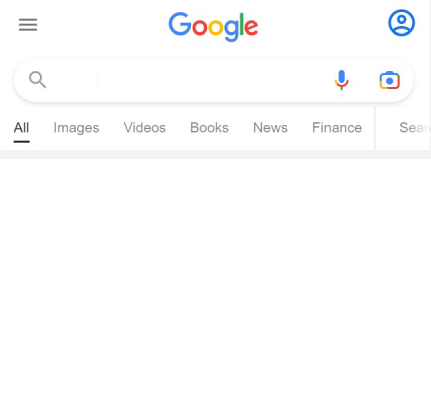The image displays a Google search page with the header bar prominently featured. Central to the scene is a horizontally oriented Google search box, which is framed by a very subtle light gray border at the bottom. Towards the right side of the page, a thin gray line is visible.

At the top center of the page sits the iconic Google logo, rendered in its signature colors—blue, red, yellow, and green. In the top left corner, three vertical gray lines are positioned, suggesting a menu icon. On the top right corner, a circular icon with a blue, blank profile picture is visible.

Beneath this area, the characteristic Google search bar is displayed with a magnifying glass icon on the left-hand side symbolizing search functionality. On the right-hand side of this bar are two additional icons: a multicolored microphone icon indicating voice search capability, and a camera icon, both in matching blue, red, yellow, and green hues.

Directly below the search bar is a navigation bar offering various search categories: All, Images, Videos, Books, News, and Finance. The "All" category is highlighted in darker gray text with a small horizontal line beneath it, indicating it is the selected filter.

In the bottom right-hand corner of the image, the word "Search" is partially visible; only "SEA" can be seen as the rest ("RCH") is cut off by the image's right border. The entire layout is surrounded by ample white space, ensuring a clean and focused interface.